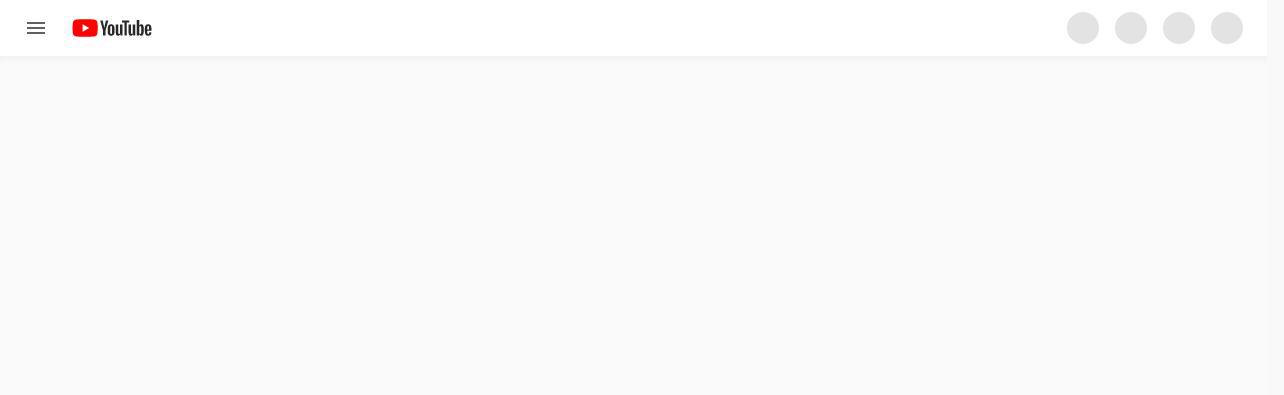The image depicts a clean, minimalist advertisement banner on the YouTube website. The background is entirely white, providing a stark and uncluttered canvas. On the far left side, there are three horizontal black lines, which are the iconic "menu" symbol indicating that additional navigation options can be accessed when clicked. Adjacent to this symbol, the recognizable YouTube logo is prominently displayed, featuring a red play button next to the word "YouTube" in black text. 

A very faint bluish-gray line runs horizontally just below the logo, subtly separating it from the content beneath. On the far right side of the banner, there are four very light bluish-gray dots aligned horizontally. Below these dots, there's a barely discernible faint bluish-gray area, which appears to outline a square, indicating an inactive or placeholder section of the website with no visible content within it.